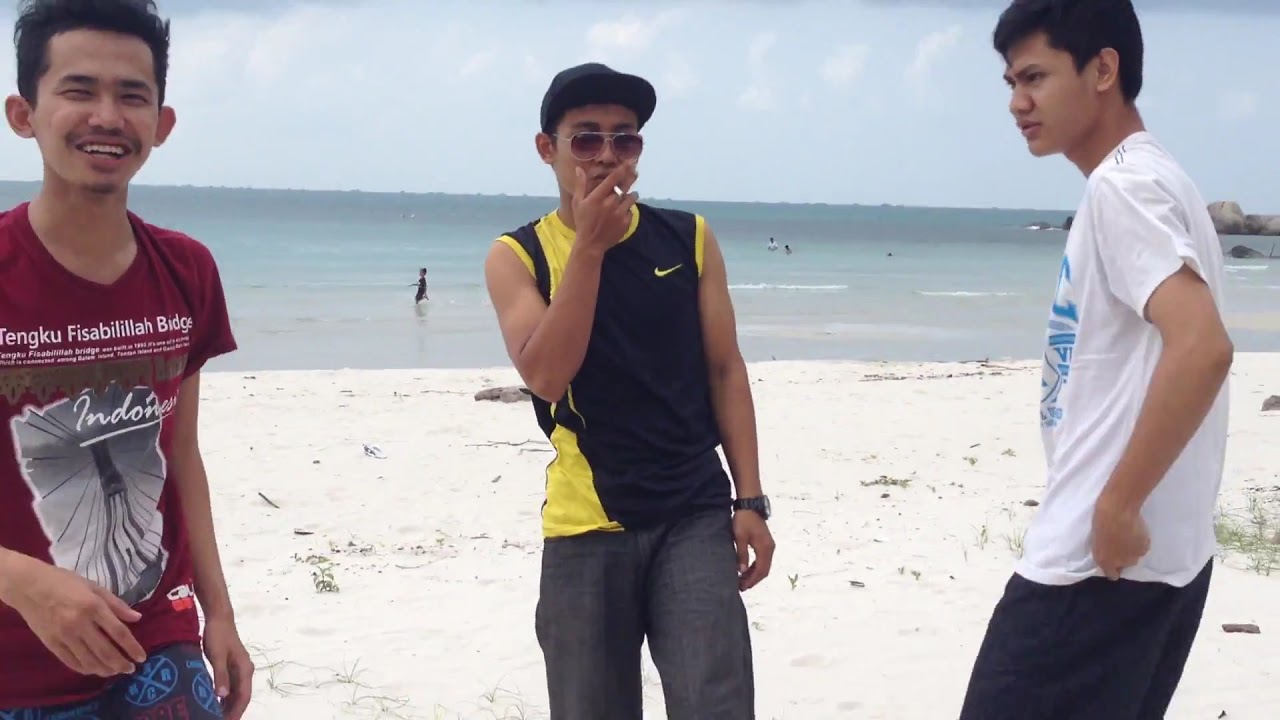In this horizontally aligned rectangular photograph taken at a beach, three men stand in the foreground, possibly friends. On the left stands a man with short dark brown hair, smiling at the camera with squinted eyes. He wears a dark red t-shirt that reads "Tengu Fisabila Bridge" with "Indonesia" written across the center, the shirt also featuring some sort of picture. The man in the middle, smoking a cigarette, sports a black cap and reddish-tinted sunglasses. His attire includes a black and yellow Nike tank top and gray pants or shorts, with a watch visible on his wrist. The man on the right, who is facing the man on the left without smiling, wears a white t-shirt with a blue print and black pants or shorts. He has short black hair and appears to be tugging at his pants. The sandy area they are standing on has small tufts of grass, and in the background lies a calm ocean with a few people in the shallow waters and further out. The sky above them is partly cloudy, filled with gray and white fluffy clouds, casting a soft light onto the scene.